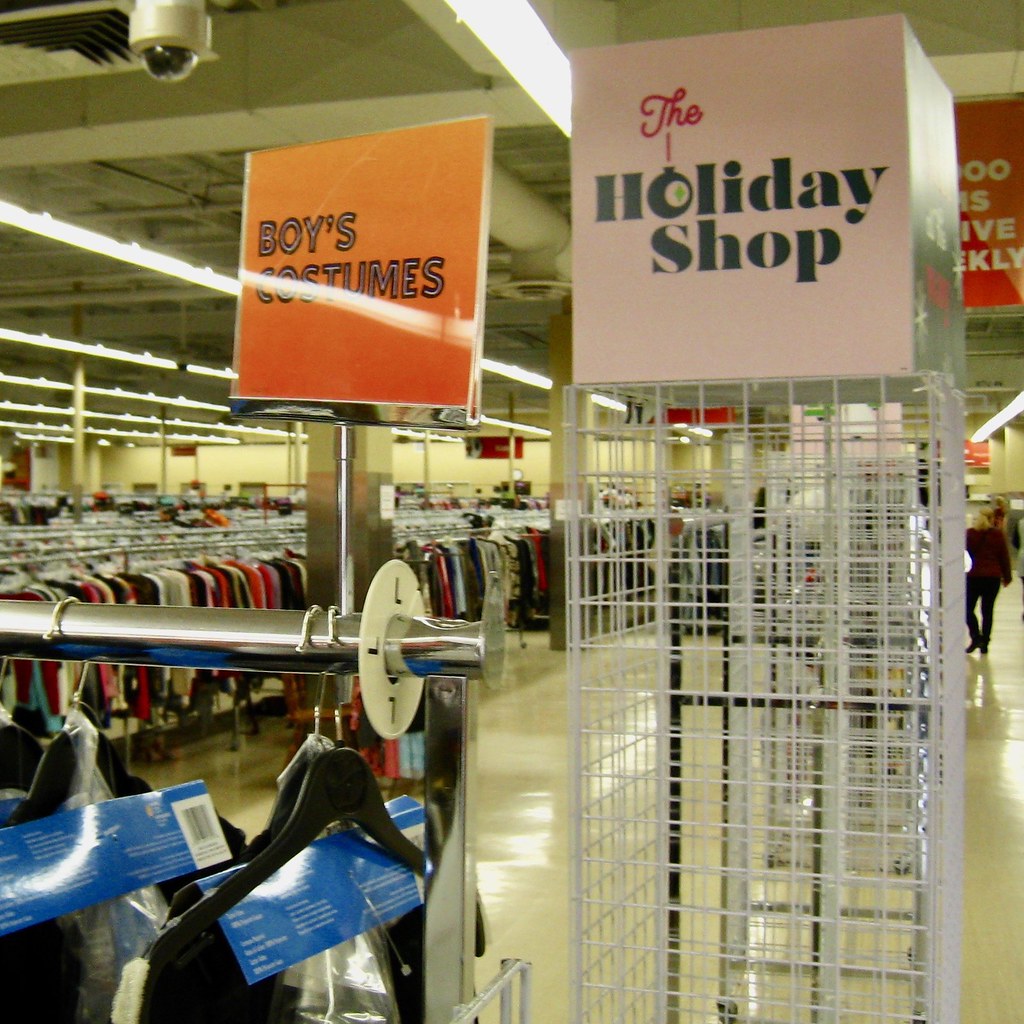The photograph captures the bustling interior of a large retail store. In the foreground, there is a large, empty white metal rack. At the top of this rack, there's a festive, holiday-themed box predominantly white with text that reads "Holiday Shop." Adjacent to this is a metal pole sign indicating "Boys Costumes" in black letters on an orange background. Below the sign, an assortment of clothing items is neatly hung on black hangers, all encased in clear plastic coverings. A white plastic disc labeled with an "L" for large is affixed to the end of the rack.

In the mid-ground, there is a long row of clothing, mostly tops and shirts, arranged on an extended rack. The floor consists of clean, white linoleum tiles. A shopper, a woman dressed in a burgundy long-sleeve shirt and black pants, is captured mid-step, facing away from the camera with one leg bent as if in stride.

Above, the ceiling features an array of track and fluorescent lighting, illuminating the entire scene with bright, even lighting. This detailed composition showcases the organized yet dynamic environment of the retail space.